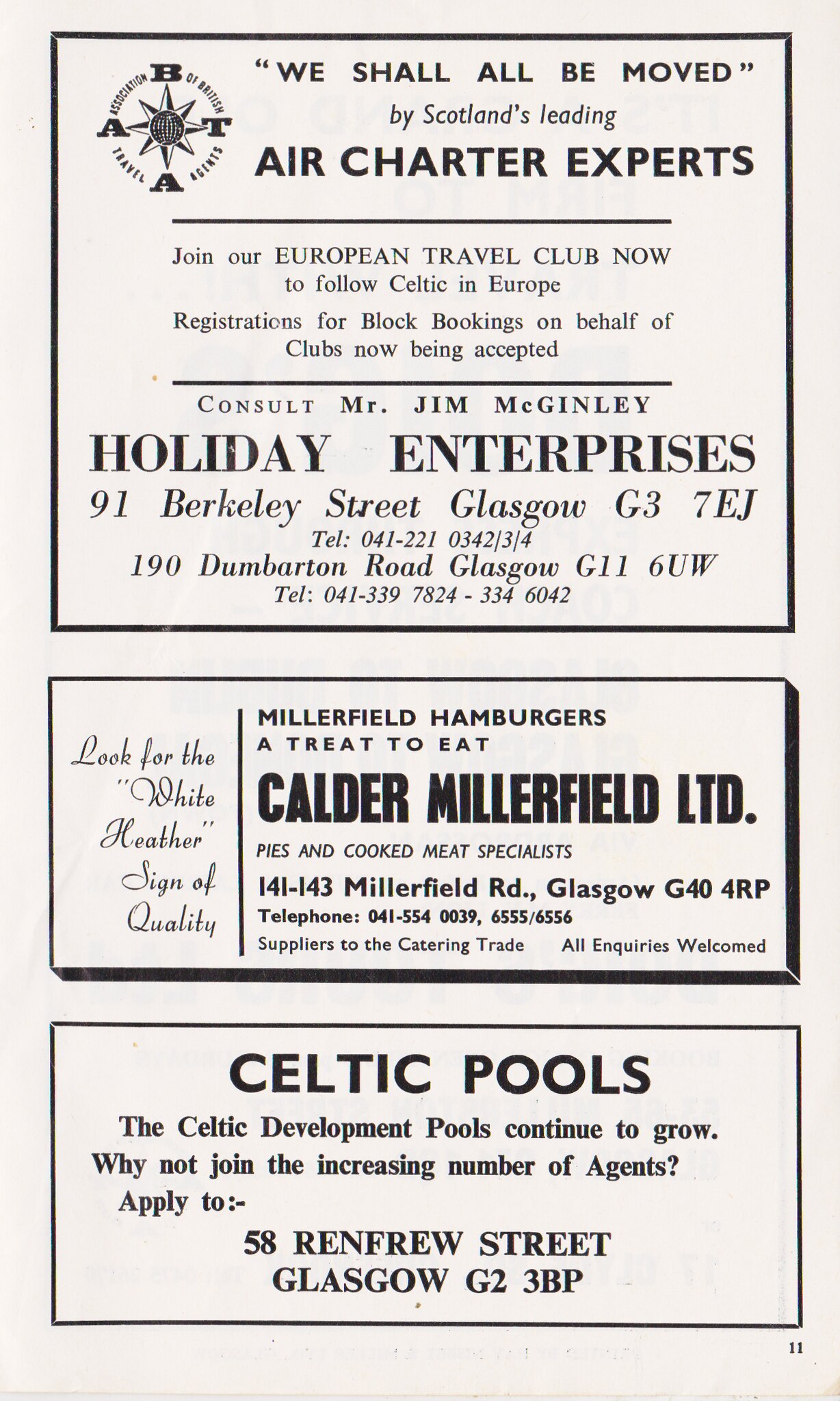The image showcases a detailed advertisement composed of three distinct rectangular sections, each promoting a different business, all set against a light blue background. In the topmost section, an image resembling the center of a compass features the letters A B T A, accompanied by the text: "We shall all be moved by Scotland's leading air charter experts. Join our European Travel Club now to follow Celtic in Europe. Registrations for block bookings on behalf of clubs now being accepted. Consult Mr. Jim McGinley Holiday Enterprises," along with their contact details. The middle section advertises "Millerfield Hamburgers, a treat to eat," produced by Calder Millerfield Limited, specialists in pies and cooked meats, followed by their contact information. The bottom section promotes "Celtic Pools," stating "The Celtic development pools continue to grow. Why not join the increasing number of agents?" with application details provided. The entire poster appears meticulously centered and well-organized, with the advertisements spaced out evenly, giving it the appearance of a magazine page marked with the page number 11 at the bottom right corner. The color scheme is predominantly off-white, black, and gray, adding a classic and formal aesthetic to the presentation.